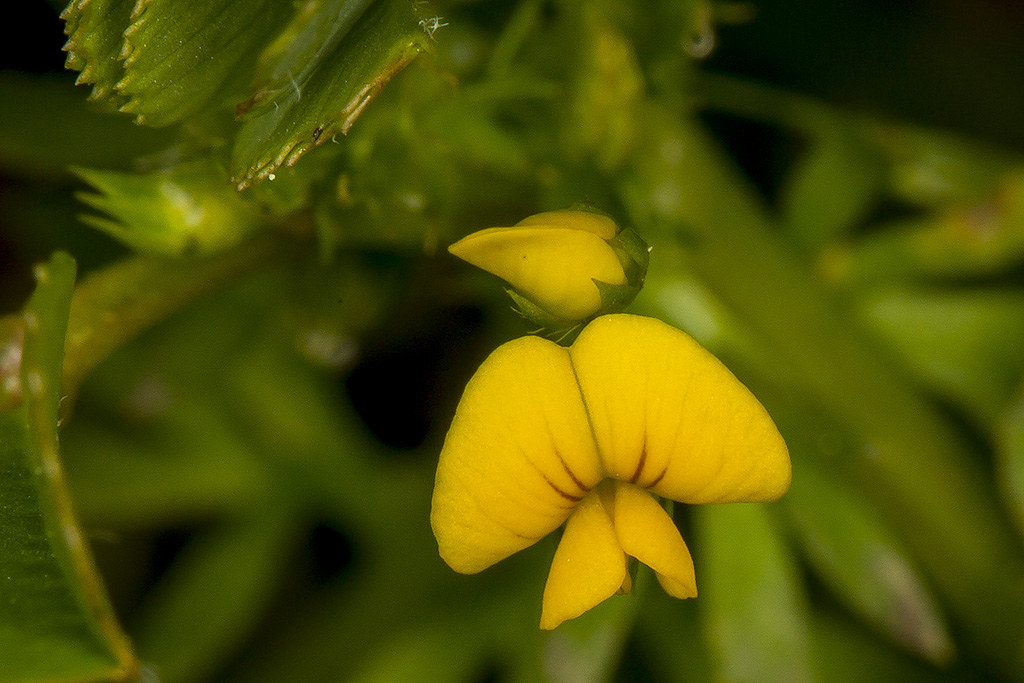A vibrant yellow flower with intricate details captures attention as it hangs upside down. The main flower features striking black and blue lines near its center, running upwards, giving it a unique texture. This central bloom also has some delicate, flimsy petals extending downward, adding to its intricate design. Just above the main flower, there is a yellow bulb encased in a green leafy cover, resembling an "M" shape with a solid base and a pronounced gray line running down the center. The plant's overall structure evokes imagery of a butterfly or moth, with its two large, wing-like petals spreading outwards and smaller petals below mimicking a bird or bug's tail. Surrounding the flower, some green leaves create a soft, blurred background, except for distinct green leaves in the upper left corner, accented with white speckles and vein-like lines descending towards the left. Each element of this flower conjures images of delicate, fluttering creatures, giving it an ethereal quality.